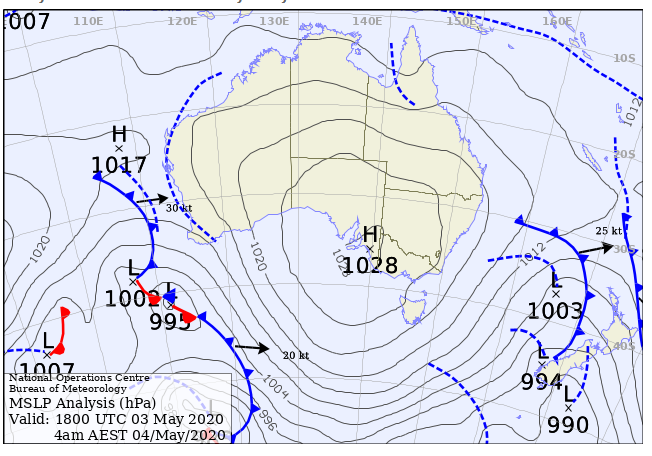The image displays a detailed weather map of Australia. The map features topographical and meteorological elements, including contour lines that indicate altitude and isobaric patterns showing atmospheric pressure. At the center of the map, a high-pressure system, marked as H1028, is located in the southeastern part of Australia. The map contains both blue and red lines with arrows, indicating the direction and flow of high and low-pressure systems respectively, with blue lines predominating. Australia's outline is highlighted in a light bluish-purple color, set against a light blue background. Additionally, the map includes intricate details such as curved and dotted lines with triangles. In the bottom left corner, there is a rectangular information box with text that reads "National Operations Center, Bureau of Meteorology," noting the MSLP analysis details and valid timing as "1800 UTC 03 May 2020 4 AM AEST 04 May 2020."